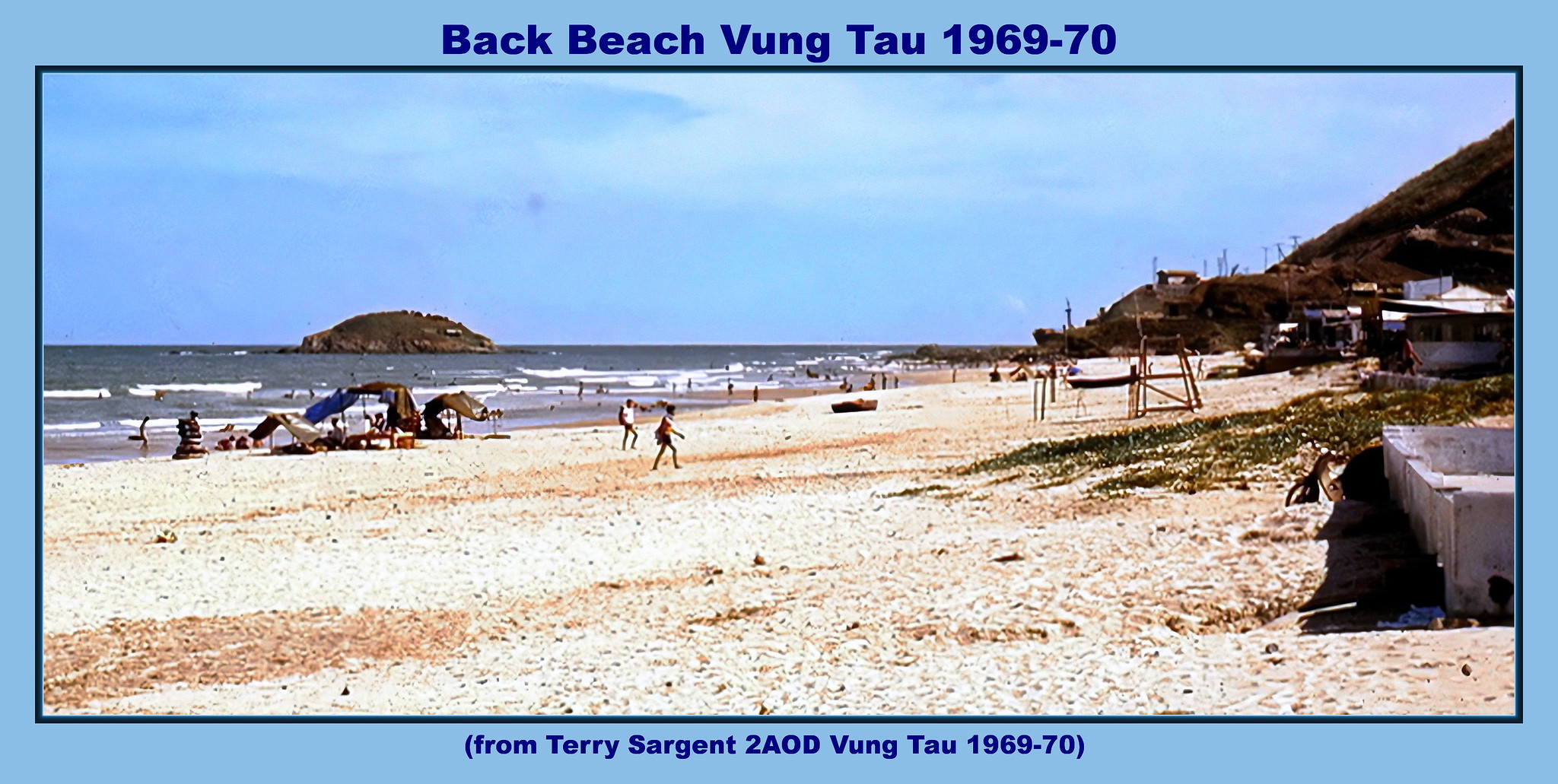This detailed photograph, likely taken in the early 1970s, captures a bustling beach scene at Back Beach, Vung Tau during the years 1969 to 1970. The image features many people scattered along the shore, with various tents, chairs, and covers visible on the sandy expanse. To the right, a small patch of green punctuates the beach, and further up are structures including buildings, fences, sheds, and dedicated areas such as a lifeguard's post. A concrete structure can also be seen near the bottom right of the image. Out on the water, an island appears relatively close, suggesting it could be easily reached by boat. The photograph, framed with a blue border, has text on the top and bottom. The top text reads "Back Beach, Vung Tau, 1969-70" in blue, while the bottom text states "From Terry Sergeant to AOD, Vung Tau, 1969 to 70," also in blue. The vintage look of the picture, along with the scene's overall ambiance, suggests it was indeed taken in the seventies.